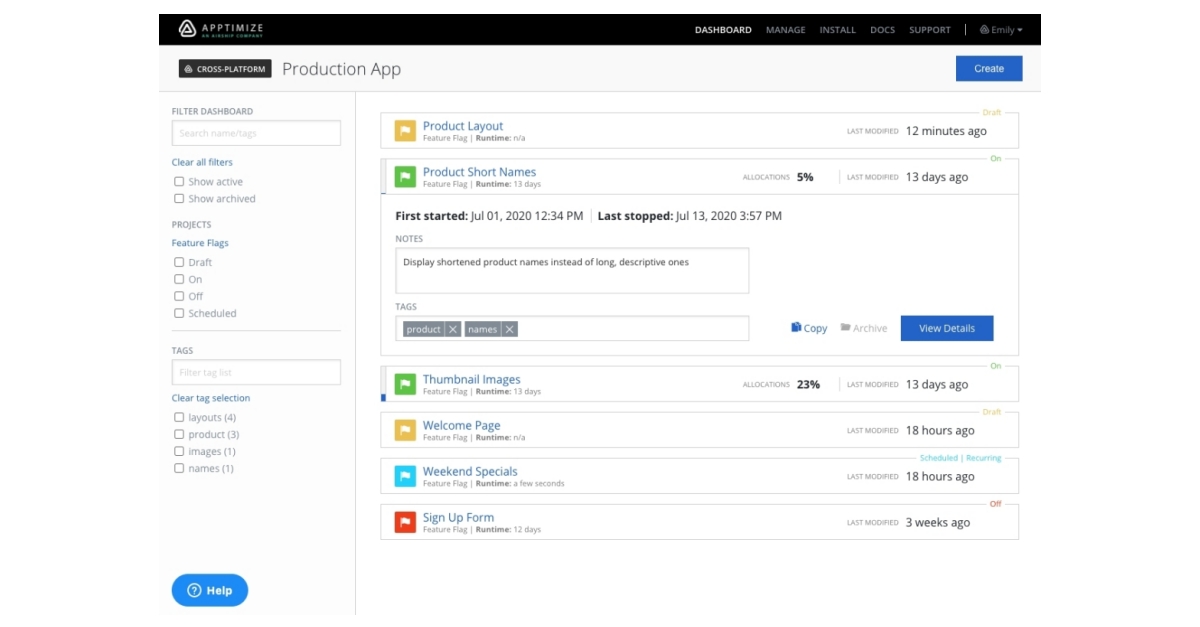Image Caption: 

The header of the page boasts a sleek black background that contrasts strikingly with the white text on the top right. Here, navigation tabs including "Dashboard," "Manage," "Install," "Docs," and "Support" accompany the user profile section labeled "Emily." On the top left, the word "Optimize" is prominently displayed next to an icon of two white, interconnected triangles.

Directly below the header, the left side contains a section titled "Cross-Platform Production App." Adjacent to this text on the top right is a prominent blue "Create" button. Below this, a comprehensive dashboard appears, beginning with filter options like "Search Name or Text," "Clear Filters," "Show Active," "Show Archived," and several project statuses such as "Feature Flex," "Draft," "On," "Off," and "Scheduled." Additional categories for refining selections include "Tech," "Layout," and "Product." None of these filters are currently checked. 

On the bottom left corner, another blue button labeled "Help" invites users to seek assistance.

Center stage on the page, green text announces a section named "Product Layout," accompanied by a yellow flag indicating a feature that was last modified 12 minutes ago. Below, a green-flagged entry labeled "Product Short Name" provides details such as "Runtime, Daily Days," an allocation of "5%," and a status last modified 13 days ago, currently marked as "On." Additional information includes the start date of July 1, 2020, at 12:34 pm and the last stopped date of July 13, 2020, at 3:57 pm. A note advises displaying shortened product names for clarity.

Lower on the page, under the section titled "Text," two items—"Product" and "Names"—are mentioned, with a blue button on the right side labeled "New Details." 

Finally, the bottom of the page features an organized list of domains and their modification dates: "Domain Images," updated 13 days ago; "Welcome Page," and "Weekend Special," both modified 18 hours ago; and a "Sign Up Form," last tweaked three weeks back.